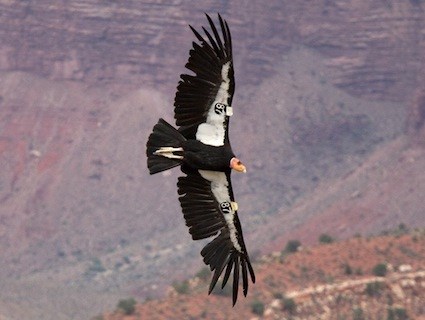In this photograph, a large bird, potentially a vulture or an eagle, is captured mid-flight with its expansive wings fully outstretched as it glides towards the right. The bird, predominantly dark in color with a white or yellowish head, features the number '87' conspicuously affixed to the underside of each wing, suggesting some form of tagging or tracking. The bird's head appears pink and bald, indicating it could be a vulture. The scene is set against a distant, blurry backdrop of a tall, rocky mountain face characterized by gray and brown tones, interspersed with patches of dirt and greenery. A subtle white streak, possibly a road, can be seen weaving through the bottom-middle to lower-right portion of the image, adding depth to the vast, rugged landscape. The photograph captures the bird in daytime, highlighting the detailed textures and colors of both the bird and the mountainous background.